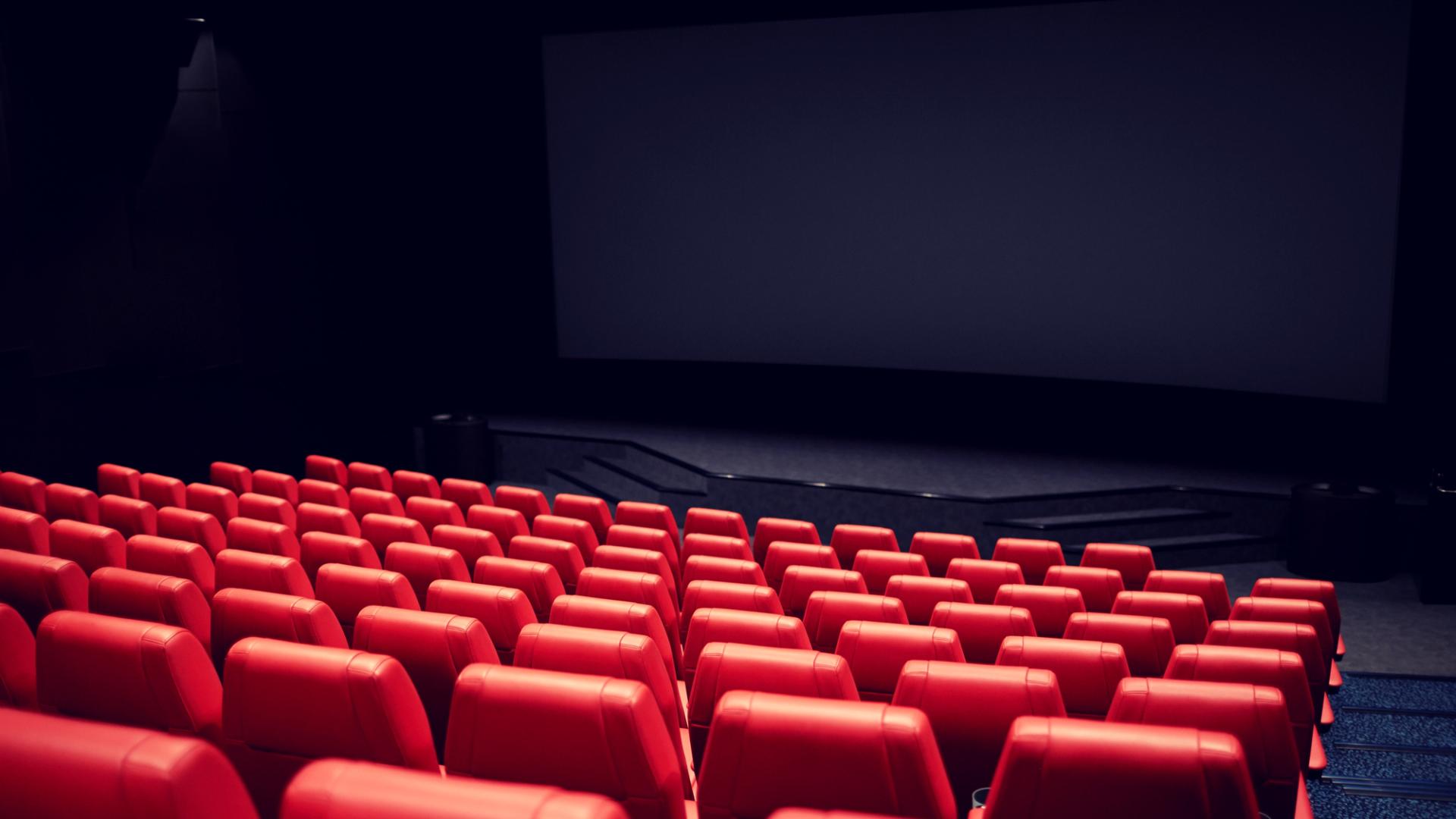The image depicts an empty theater from an elevated perspective, capturing a scene that combines elements of both intimacy and grandeur. The focus is towards the stage, which is covered in black flooring and backed by a black wall, devoid of curtains or additional scenery. Each side of the stage is flanked by black stairs leading up to it, adding to the sense of symmetry and structure.

The seating area stretches out in front of the viewer, revealing rows of bright red leather seats. The visible portion includes approximately seven to ten rows, each consisting of about 14-16 seats across, though the precise number is difficult to ascertain due to the shadows and angles. Despite the overall darkness, the overhead lights suspended above the seating area provide enough illumination to outline the seats and faintly reveal the stage.

Notable for its lack of modern movie theater amenities, the theater resembles more of a lecture hall or a venue suited for events like TED talks, giving it an educational rather than entertainment-focused atmosphere. The left side of the image fades into darkness, while the right side features blue shades and a staircase, suggesting additional ascending pathways. The overall ambiance is one of quiet anticipation, imbued with the potential for performance or presentation.